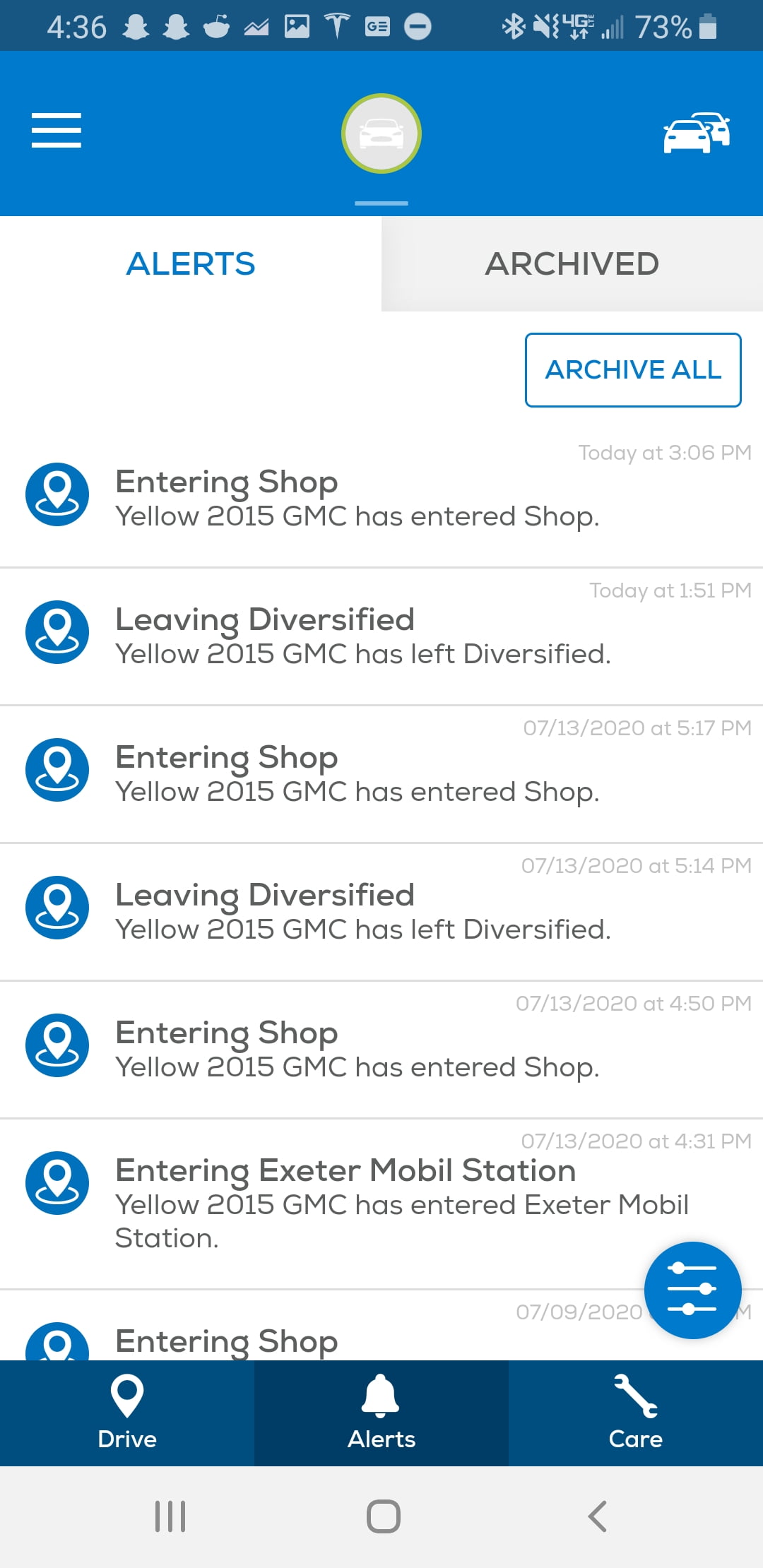This screenshot, taken at 4:36, showcases the interface of a mobile application featuring various status alerts related to a yellow 2015 GMC vehicle. The top of the screen shows essential system icons including two white Twitter ghost icons, a Reddit alien icon, a Tesla insignia, the Bluetooth symbol, a two-bar carrier signal, and a battery life indicator at 73%. Notification sounds are turned off, as indicated by the relevant icon.

At the top, there's a blue banner with a gray circle housing a vehicle icon. Adjacent to this icon on the right are two staggered vehicle icons. The "Alerts" tab is highlighted in blue text, while the "Archived" tab is inactive and displayed in gray. There is also an "Archive All" button in blue text.

The main section lists activity alerts for the yellow 2015 GMC. The first entry notes "Entering Shop," indicating that the vehicle has entered the shop. This is followed by a log reading "Leaving Diversified," noting that the vehicle has left a location named Diversified. The final entry repeats the "Entering Shop" status update for the same vehicle.